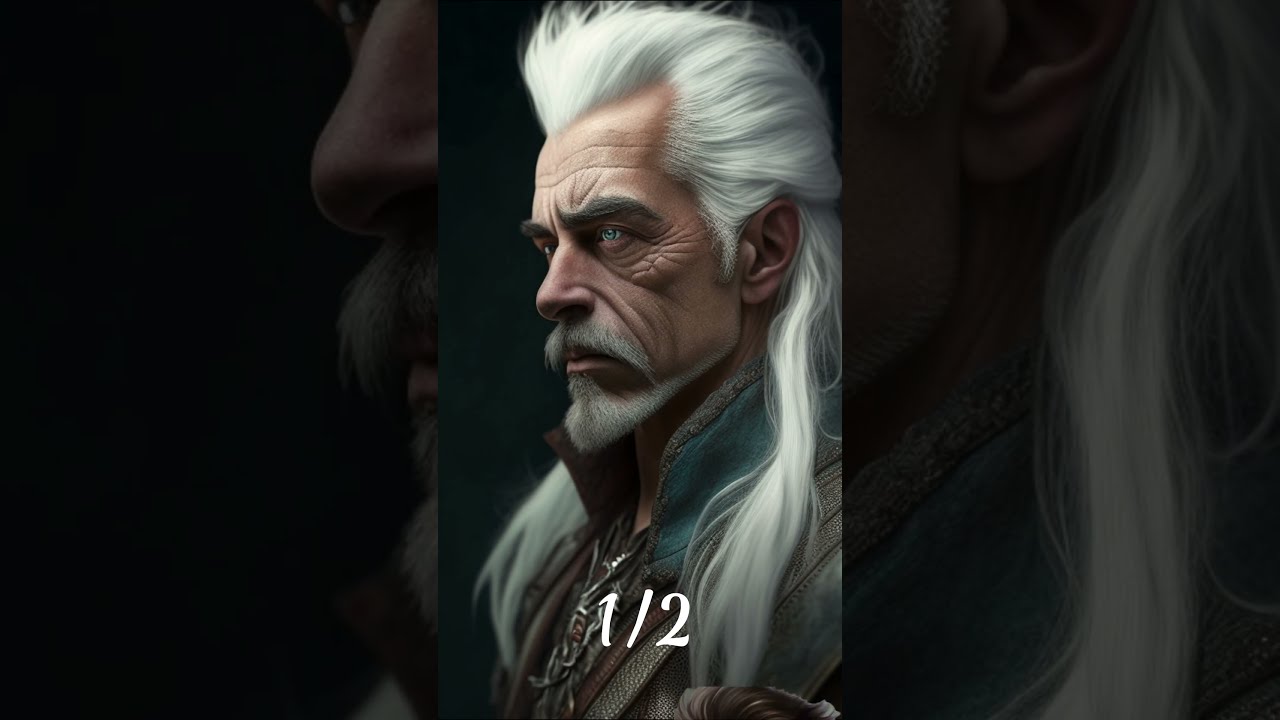The image portrays a detailed AI-generated character, potentially from a fantasy world or video game. The subject is an older, battle-hardened man with striking long white hair flowing past his shoulders, a chiseled jaw, and a well-trimmed gray mustache and small beard. His face is marked with wrinkles that add to his fierce and determined expression. His piercing blue eyes, intense and slightly scowling eyebrows, suggest a life of many battles. The man is adorned in a high-collared blue tunic paired with a possible leather vest or armor, and he wears an amulet necklace, emphasizing his mystical or warrior persona. The image is vertical, showing a side profile up to his shoulders and chest. At the bottom, there is white text that reads "1/2" or "1 of 2."